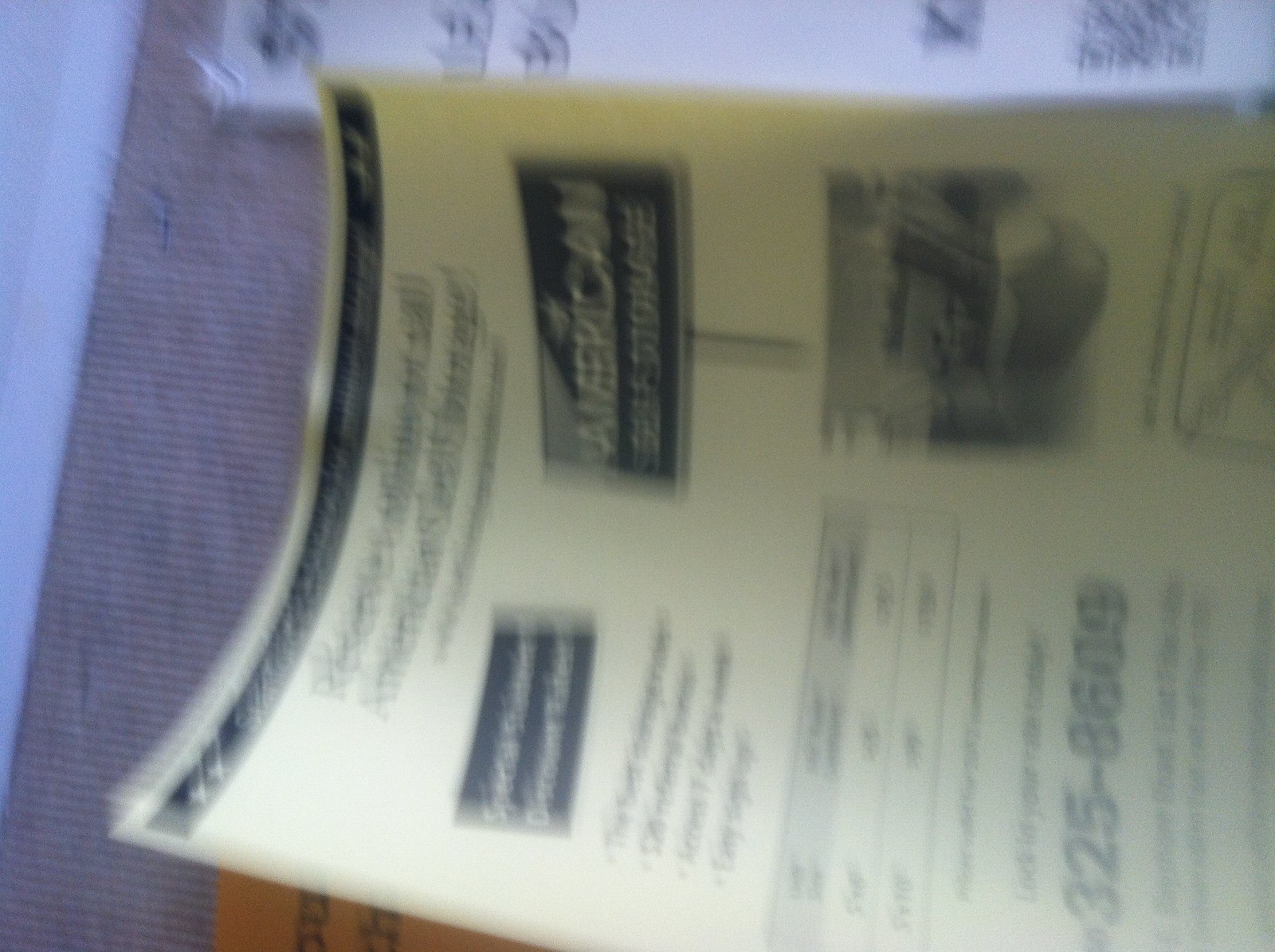This color photograph is a close-up shot of a somewhat indiscernible scene, with blurred elements that make identification challenging. On the left side, there is a blue edge that hints at some sort of structure or object. Below this, a surface—possibly a brownish floor or table—can be seen. Dominating the upper section of the image is a piece of paper with black text. The focal point of the photograph is a large, yellowish paper centrally located and oriented at an angle requiring a tilt of the head to the left for clearer viewing. Despite the blur, the paper displays black writing and features black rectangles. The rightmost black rectangle resembles a sign, marked with the word "American" at the top. The bottom part of this rectangle includes an indistinct photograph, seemingly depicting a bowl, potentially containing food or flour. Below and to the left of this setup, part of a phone number is visible in large black numerals.